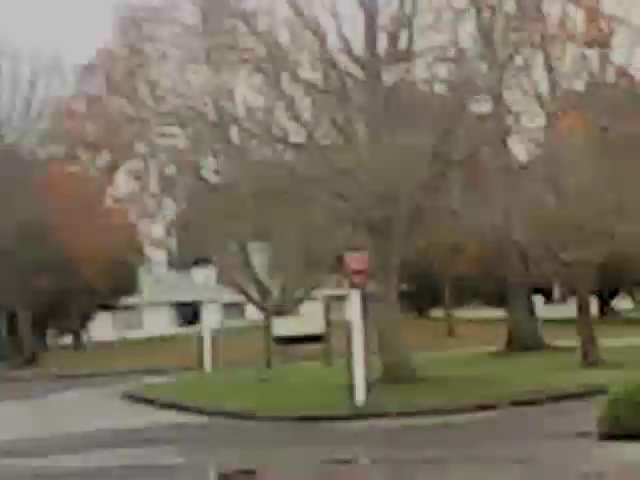This photograph, taken outdoors likely in the late afternoon with overcast skies suggesting impending dusk, captures a multifaceted scene. In the distant background, a white building stands, bordered by patches of green and tan grass. Flanking the edges of the image are trees adorned with vivid red leaves, indicating the vibrant hues of the fall season. Prominently in the foreground, a gray roadway spans the image, interrupted by a plot of green grass peppered with various trees—some boasting autumnal red foliage and others stripped bare of leaves. At the forefront of this grassy area, a white post topped with a conspicuous red object further adds to the composition, juxtaposed against another stretch of gray roadway laid out at the very front of the frame.